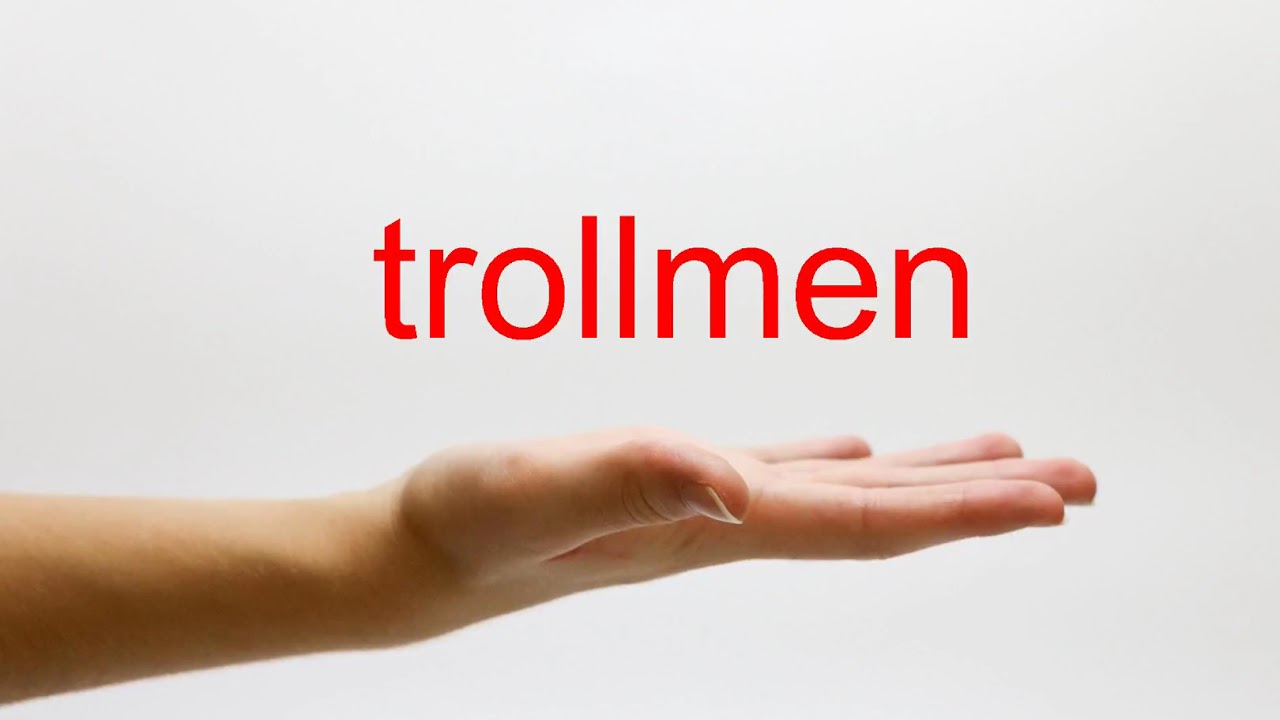The image features a background in a light gray or white tone. Dominating the scene is a small-font, red text reading "trollmen" (spelled T-R-O-L-L-M-E-N with all lowercase letters) positioned close to the top center horizontally and occupying the middle section vertically. Below this text, a right hand with light skin extends palm-up from the bottom left towards the center-right of the image, reaching approximately 70% across the width of the frame and occupying the lower 25-30% of the visual space. The hand is oriented with the thumb closest to the viewer, enhancing the sense of depth. The main colors in the image are the neutral gray background, the light skin of the hand, and the vivid red of the text.